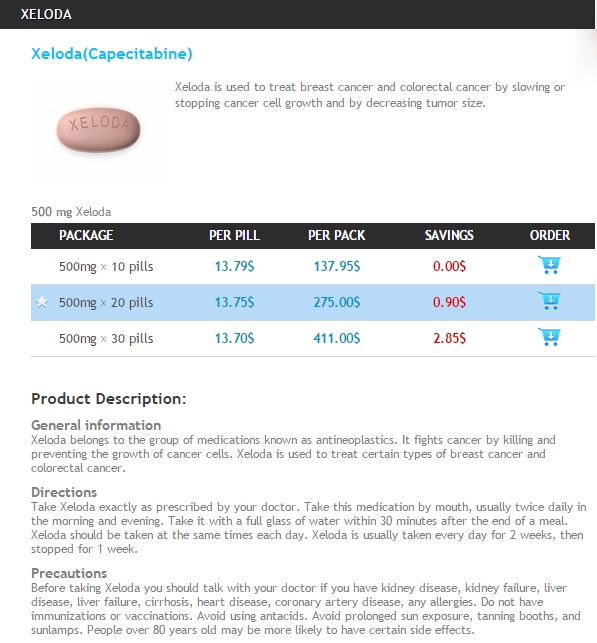This screenshot captures detailed information about the medication XELODA. At the top of the page, "XELODA" is prominently displayed in a black bar with white font, and this is followed by the chemical name "Capecitabine" spelled out in blue font in parentheses. An image of the pill is featured, showing its oval shape and the imprint "XELODA" on its surface.

The accompanying text explains that XELODA is used to treat breast cancer and colorectal cancer by slowing or stopping the growth of cancer cells and reducing tumor size. The dosage described is 500 milligrams. Pricing information is divided into sections based on quantity: 
- For 10 pills, the cost is $13.79 per pill, totaling $137.95 per pack.
- For 20 pills, the cost is $13.75 per pill, totaling $275.00 per pack.
- For 30 pills, the cost is $13.70 per pill, totaling $411.00 per pack, offering a savings of $2.85.

Below this, additional sections include a product description, general information, directions for use, and a paragraph detailing precautions to be taken while using the medication.